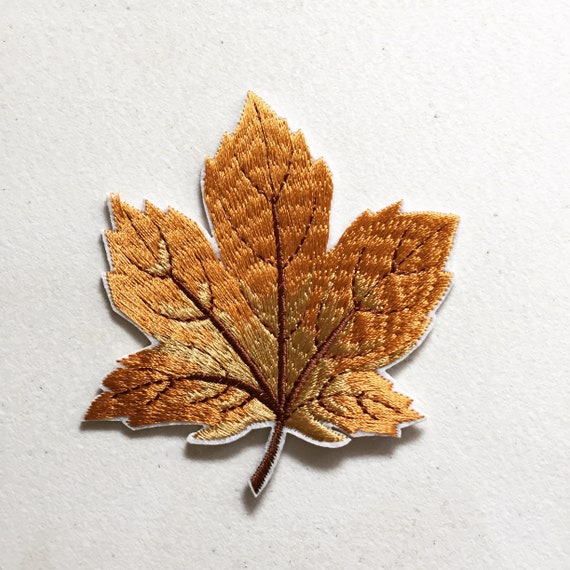This photograph features a detailed, embroidered patch designed to be sewn or ironed onto fabric. The patch, intricately crafted to resemble a maple leaf, is set against a white background, creating a subtle shadow that highlights its 3D quality. The leaf, evocative of autumn, showcases five distinct points, with colors ranging from dark amber to various shades of brown, including tan and medium brown. The main stem is dark brown, branching out into smaller veins within each section. These veins branch further, emphasizing the leaf's texture. The patch outlines with a clean, white border, enhancing its definition. The leaf's jagged edges and the transition of colors across its surface capture the essence of fall foliage, making it a striking and lifelike representation.